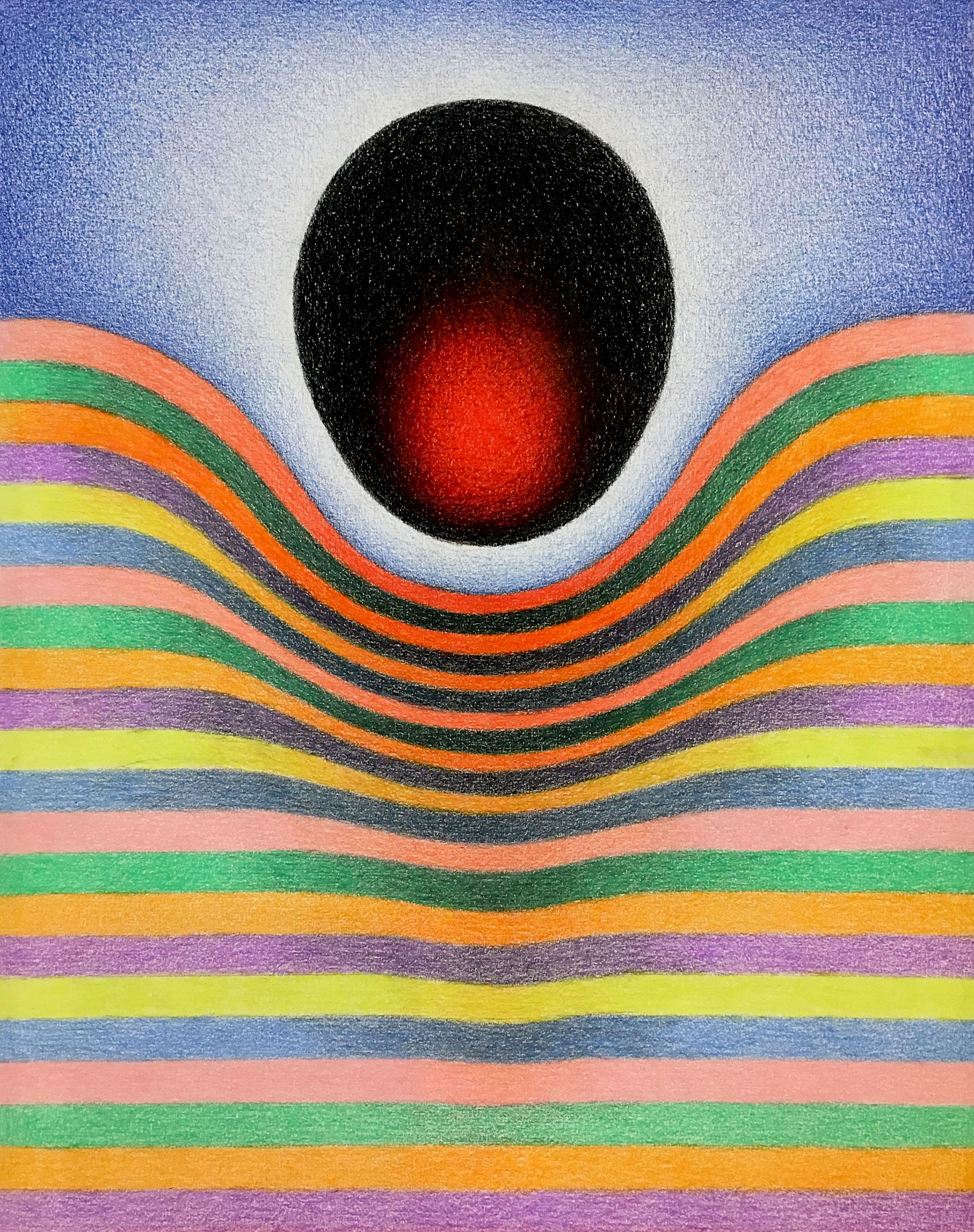This is a detailed hand-drawn illustration using colored pencils. The artwork is abstract, dominated by a series of thin, multicolored horizontal stripes that ascend from the bottom of the image to the center. These stripes follow a recurring sequence of colors: purple, orange, green, pink, blue, and yellow. Initially straight, the lines start to bend and curve near the center, responding to an unusual effect created by a central object.

The central object is a dark, blackened, egg-shaped or oval form situated in the upper middle of the image. This object has a glowing bright red section near the bottom, resembling a dot or light. The object's presence seems to exert a kind of gravitational pull on the stripes below, causing them to warp around it, creating a valley-like effect as they approach and bend around this shape.

Surrounding the central black object is a gradient background that transitions from white around the object to a grainy blue at the top, adding depth and contrast to the illustration. The blue tone is interspersed with white specks, enhancing the textured appearance of the background. Overall, the image conveys a sense of dynamic interaction between the vibrant horizontal lines and the enigmatic central shape, creating a vivid, swirling abstract composition.